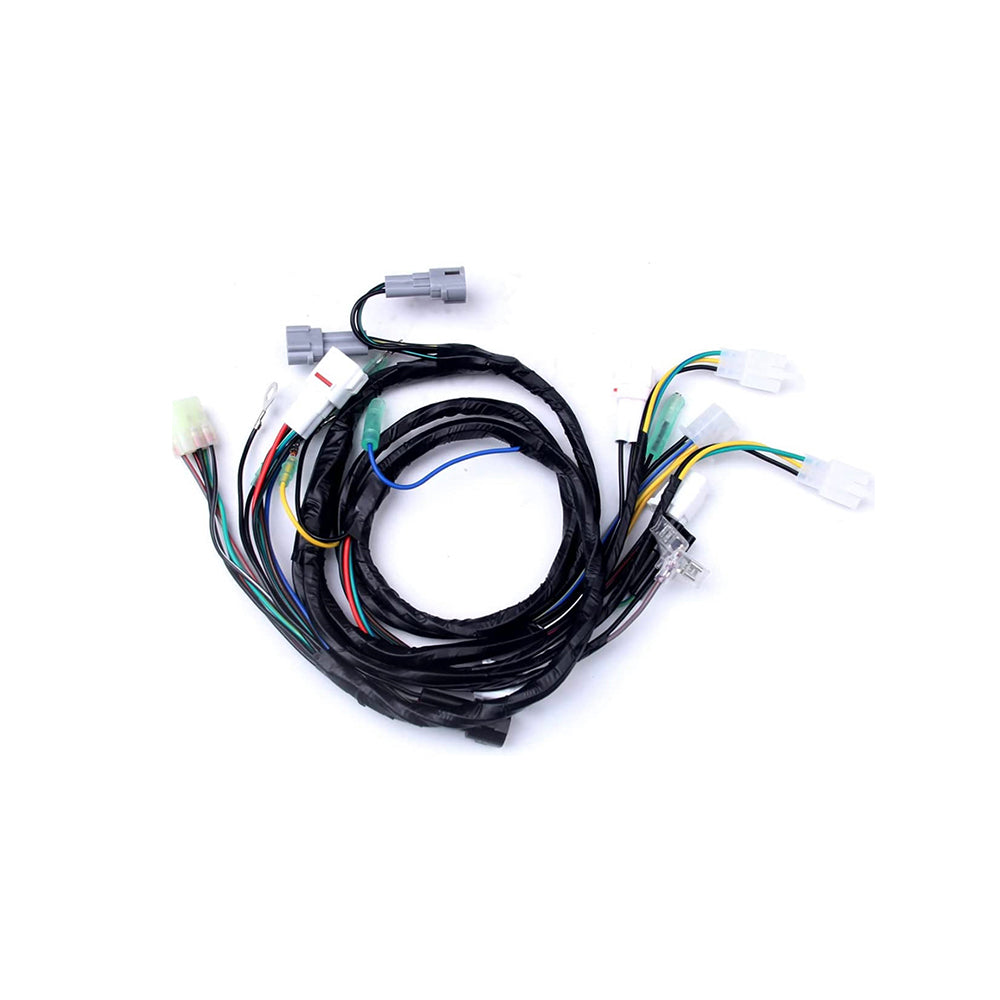The image depicts a coiled set of black cables, some appearing frayed with exposed inner wires in a range of colors, including yellow, blue, navy blue, green, orange, and red. These inner wires are intricately intertwined and some are partially wrapped with black electrical tape to keep them intact. The cables feature various connectors at their ends, resembling the type used for connecting old-fashioned phone plugs to wall outlets. The connectors come in different colors: predominantly white, with some gray and even a turquoise connector. The entire coil is artistically photographed against a white background, highlighting the vivid, intertwined wires and their connectors.